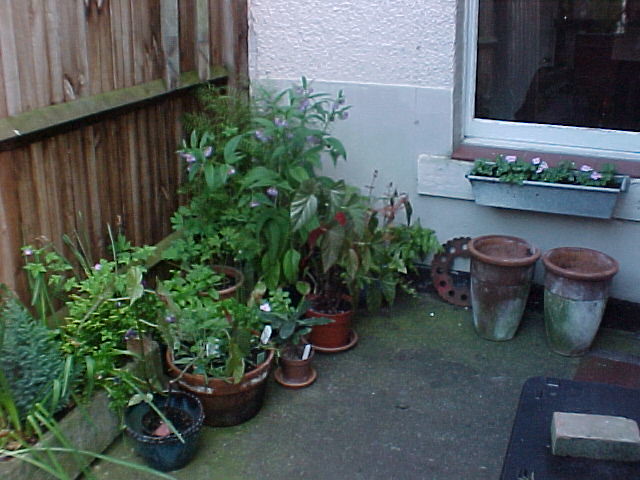The photograph captures a quaint corner of a patio or backyard brimming with potted plants set on a stone ground. To the left, a weathered wooden fence, possibly water-damaged, adds rustic charm, while various pots line the area, including a striking concrete planter with a lush flowering plant. Towards the front, there's a large square dirt patch with a small tree growing from it. On the right side, a metal gear leans against a building wall, itself adorned with a window situated above the scene. Directly beneath the window, a windowsill holds a potted plant with pink flowers, adding a pop of color. Below this, two empty terracotta pots rest on the stone ground. Scattered around are pots of different sizes and colors, mostly red with a few black ones, housing an array of plants. Some pots even have white markers identifying the plants, and there’s a mix of herbaceous greens and taller sticks. In the lower right corner, a brick and a blue plastic tote lid make a modest appearance, contributing to the eclectic ambiance.